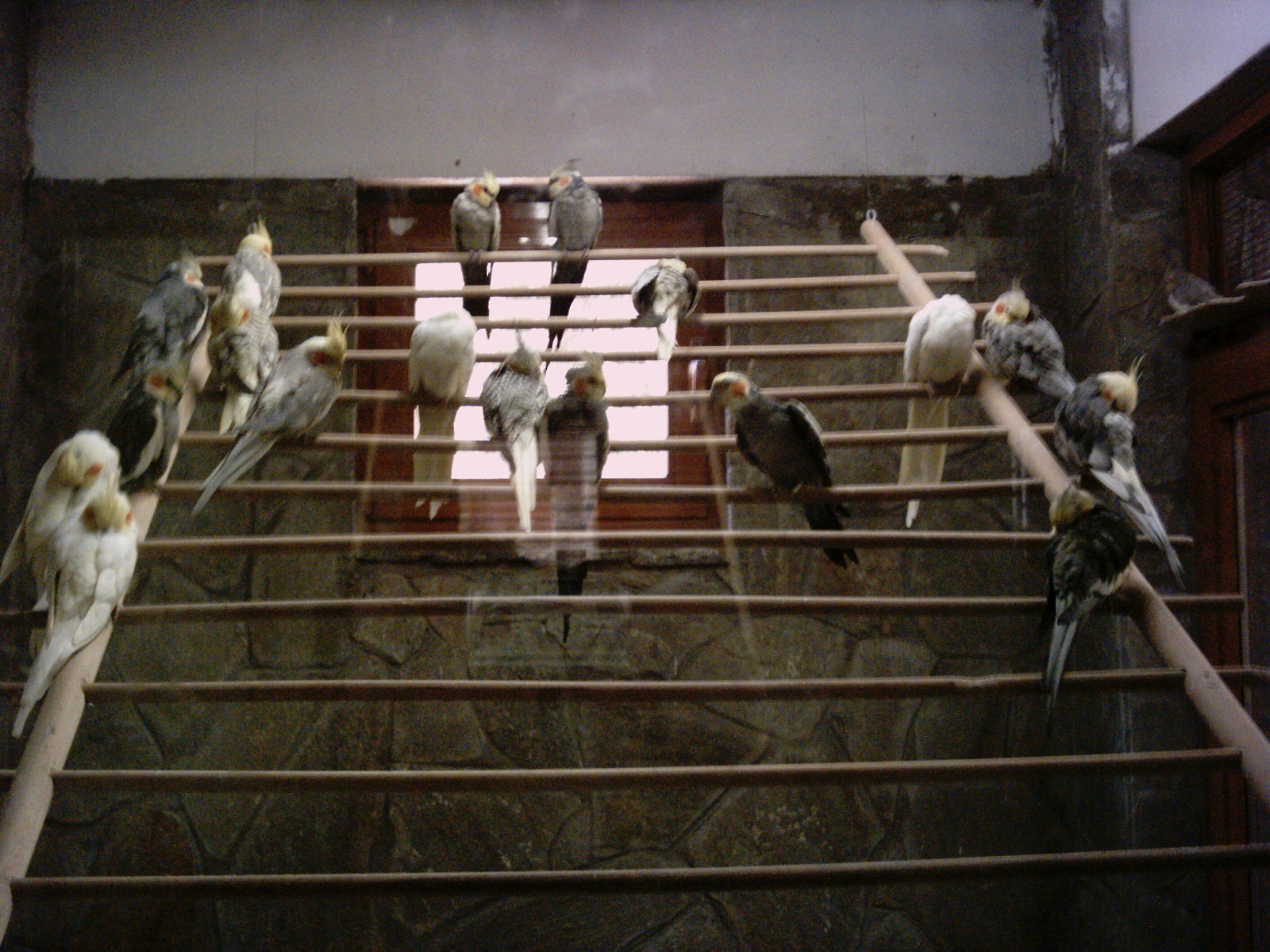The color photograph captures an interior setting, potentially a pet store, aviary, or even an attic, featuring a rack that resembles a wooden ladder diagonally positioned against a stone and white wall. The stone wall is composed of browns and grays, while the upper section includes a white wall and a window with a red wooden frame. The rack, made of thick wooden sticks on the sides connected by thinner sticks, hosts around 15 birds. These small parrots include a mix of gray, white, and some brownish bodies, with many of them displaying distinctive yellow heads. The birds are perched at various points across the rack, including several in front of the window. A bird is also noted on the right-hand side of the setup.